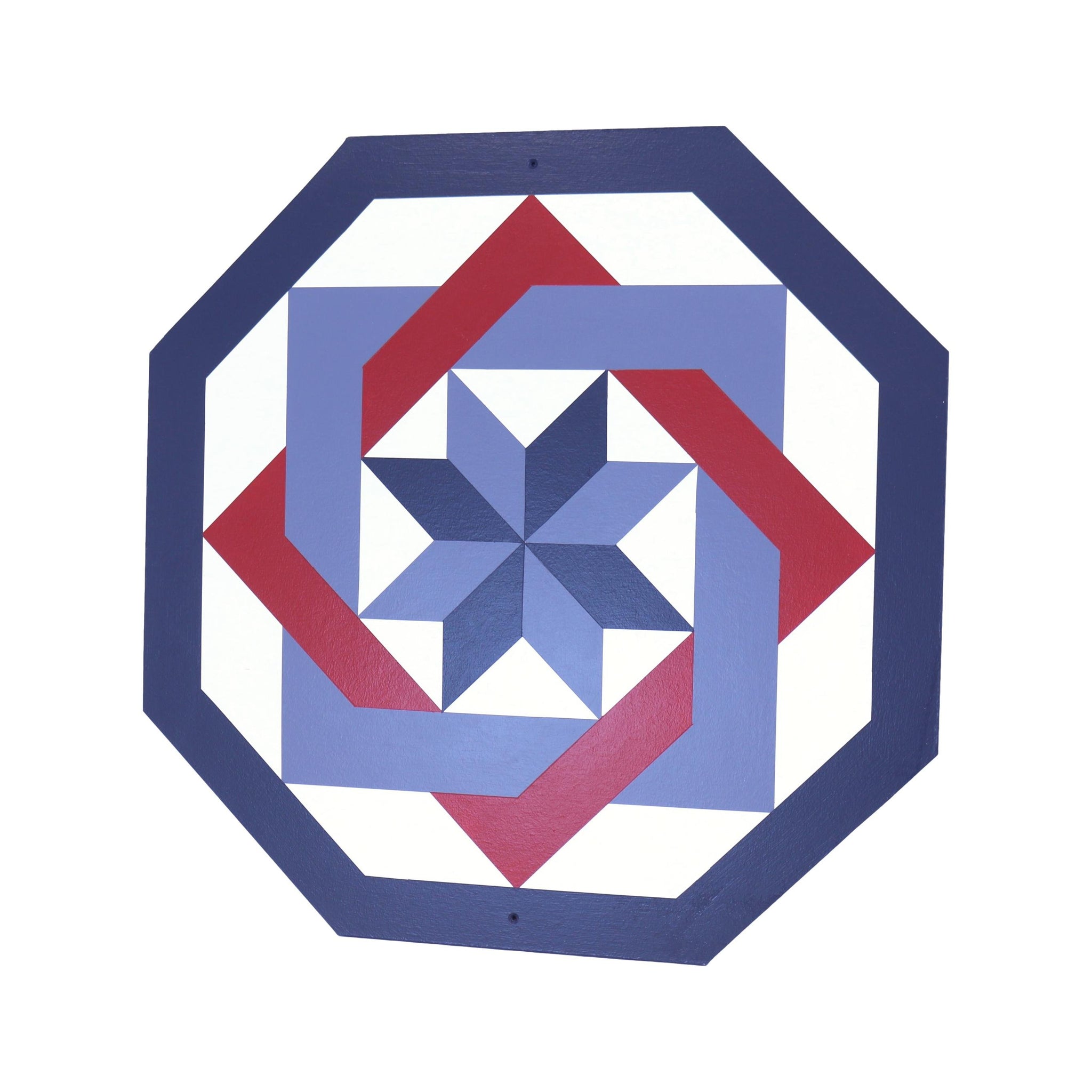The image depicts a purple octagon on a white background. Inside the octagon, there is a light blue square, and within this square, a dark red (oxblood) square is rotated to resemble a diamond. At the center of the squares, a complex star shape is formed by overlapping light blue and dark blue triangles. The star creates an optical illusion with its intricate triangular patterns pointing towards the center. The octagon itself has a dark blue border and appears slightly tilted. The overall composition is a striking interplay of geometric shapes and colors.